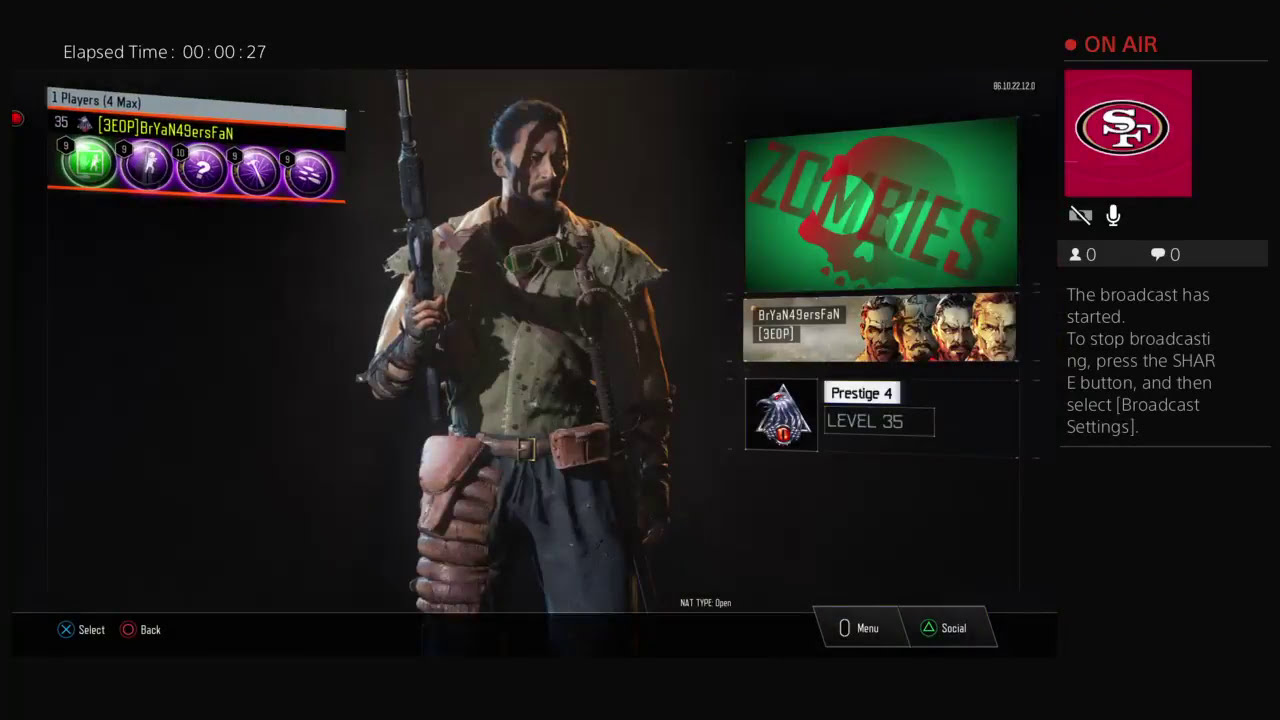The image depicts a dark screen from a video game, likely "Call of Duty," featuring a central animated character in rugged attire. The character wears a cutoff shirt, a pair of goggles around his neck, and a holster, holding a shotgun in his right hand that extends upwards. His pants are tattered blue, and he has dark features with a downward gaze to the right, casting a shadow across his face from the gun. To the left of the character is a series of circles, with the first one green and the next four purple, titled "Players 1/4 Max." The top left corner shows the elapsed streaming time, "00:00:27". 

To the right of the character, a green screen displays the word "Zombies" in red letters, with a small rectangle below it showing the faces of different characters. Below this, a box states "Prestige 4 Level 35." 

In the far right corner, a red "On Air" indication is accompanied by the San Francisco 49ers icon, followed by broadcast information, "The broadcast has started. To stop broadcasting, press the Share button, then select Broadcast Settings." At the bottom of the screen, control options are listed: "X: Select," "Circle: Back," "Start: Menu," and "Triangle: Social."